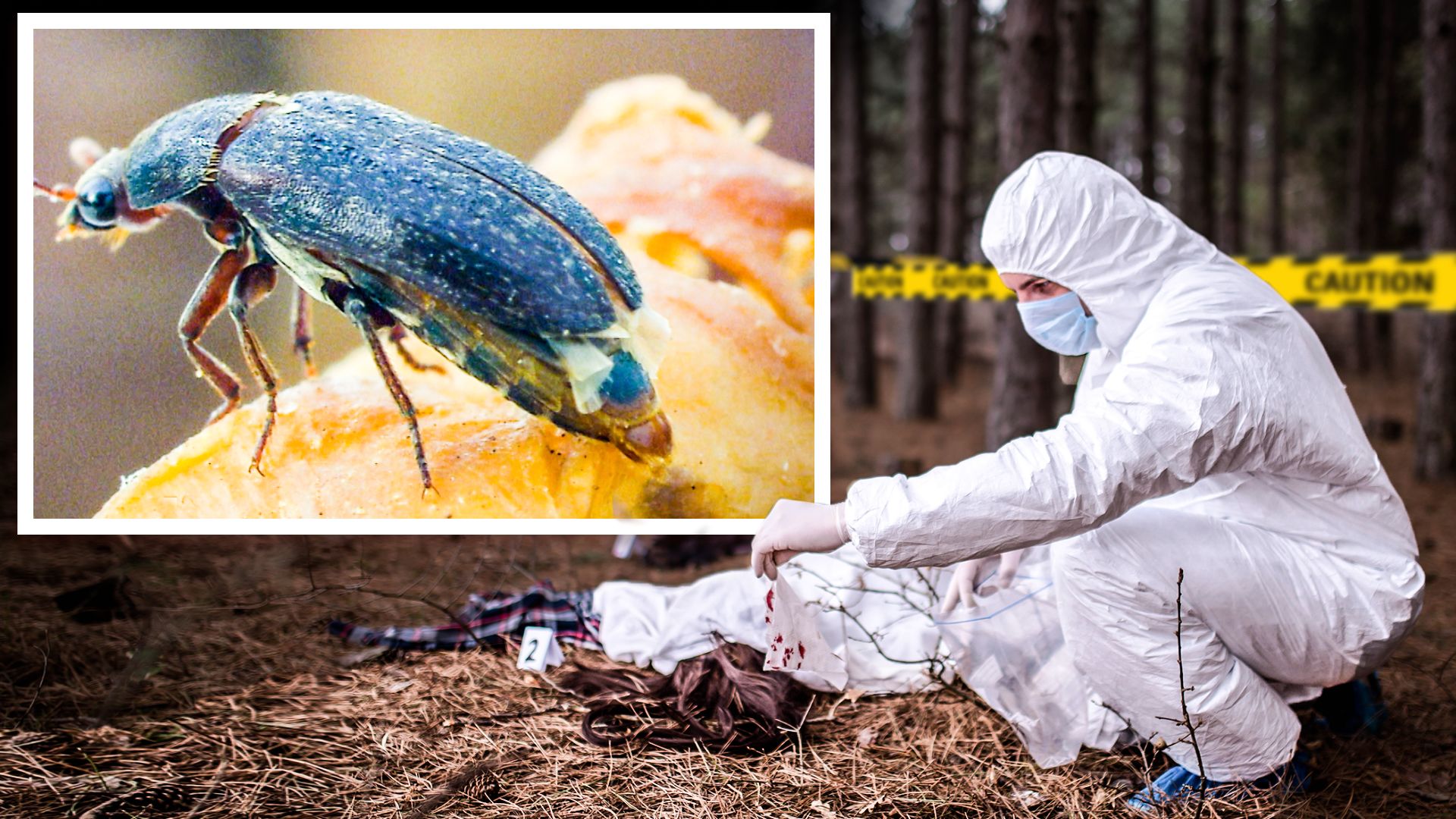The image depicts a man dressed in a white hazmat suit, seated atop a dirt hill interspersed with weeds and brown sticks. He is wearing a light blue COVID mask and off-white rubber gloves, suggesting he is engaged in some sort of decontamination or forensic activity. The focal point of his attention appears to be a body covered in white sheets with visible bloodstains and a head of thick brown hair protruding from underneath, hinting at a possible crime scene. Marking the scene is a small placard with the number '2' next to the body. Enhancing the complexity of the photo is a rectangular inset on the top left corner, outlined in yellow, featuring a close-up of a bluish-black insect, possibly a beetle or roach, on a yellow surface. This reinforces the forensic theme, as the image within the image expands horizontally to the middle and vertically to the bottom third of the main picture. The surrounding area includes a straw-covered forest floor and tree trunks in the background, bordered by yellow caution tape forming a perimeter.